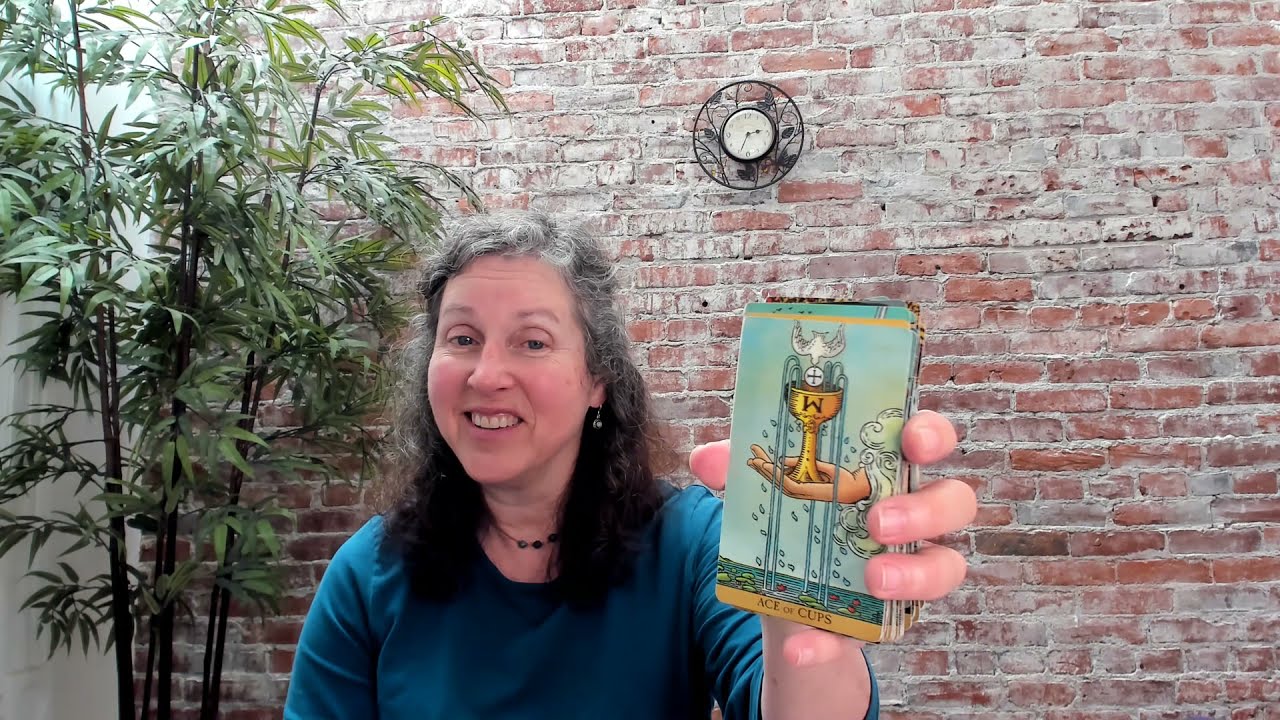In this detailed photograph, the primary focus is a smiling woman, likely in her 40s or 50s, with long, gray-to-black ombré hair cascading past her shoulders. She has a peach fair complexion and is dressed in a light blue long-sleeved shirt, with the sleeves slightly pushed up to reveal her forearm. Her attire is complemented by a matching blue necklace. The woman is positioned off-center to the left but remains the main subject of the image. She extends her left hand forward, prominently holding a vividly colored booklet, which is adorned with gold, blue, red, and green hues. The booklet's cover features an intricate illustration of a golden chalice with water and a white bird, along with the text "Ace of Cups" at the bottom.

Behind her, the scene is set against a faded red and gray brick wall, indicating an indoor setting. Over her right shoulder (the viewer's left), a plant with slender stems and leafy greens is visible, adding a touch of natural greenery to the composition. Further enhancing the background, a small black and white clock, showing the time as approximately 2:35, is affixed to the brick wall. The overall image captures a moment where the woman appears to be presenting or showcasing the booklet, possibly tarot cards, in a clear and inviting manner.